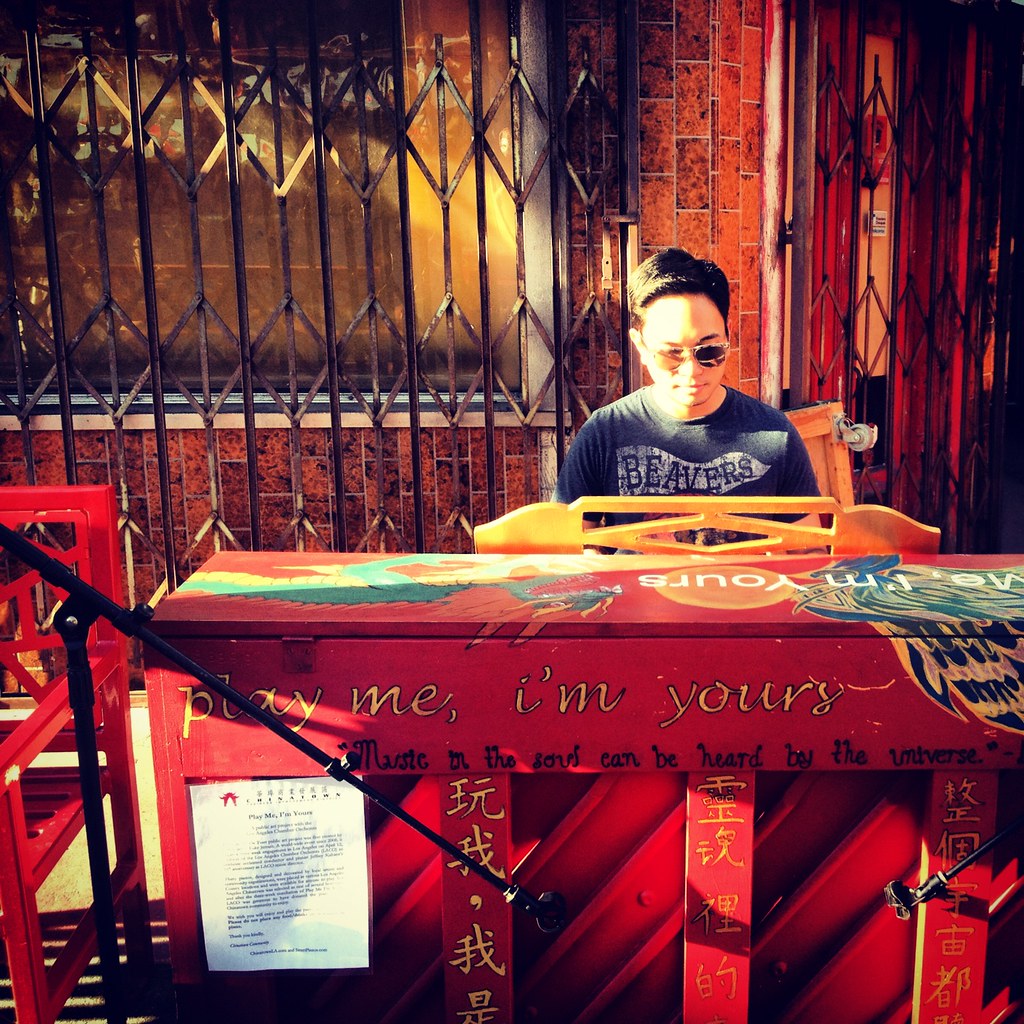In this vibrant street scene, a colorful piano adorned with red, blue, green, yellow, and white colors sits on the sidewalk, catching the eye with the yellow text "Play me, I'm yours" and "Music of the soul can be heard by the universe" prominently displayed on its surface. The piano is situated in the bottom third of the image, slightly to the right, and features a laminated paper, possibly with more details or music, affixed to it. A black microphone stand is positioned towards the left of the piano, ready for amplification. On the left side, a red-painted bench or chair adds to the vivid color palette against the backdrop of a red brick wall, which includes doorways covered by folding steel doors. 

A young Asian man with black hair, wearing tan sunglasses and a blue t-shirt that says "Beavers," is seated at the piano, absorbed in playing the instrument. His position is central, right above the piano, highlighting his engagement with the music. The scene is encased by various elements: a dark fence directly behind the player, a window to the left of the piano, and additional visual interest from the brick wall and doorways to the right. The entire setup suggests a public art installation designed to invite passerby participation, bringing music into the urban fabric and emphasizing interaction with the community.